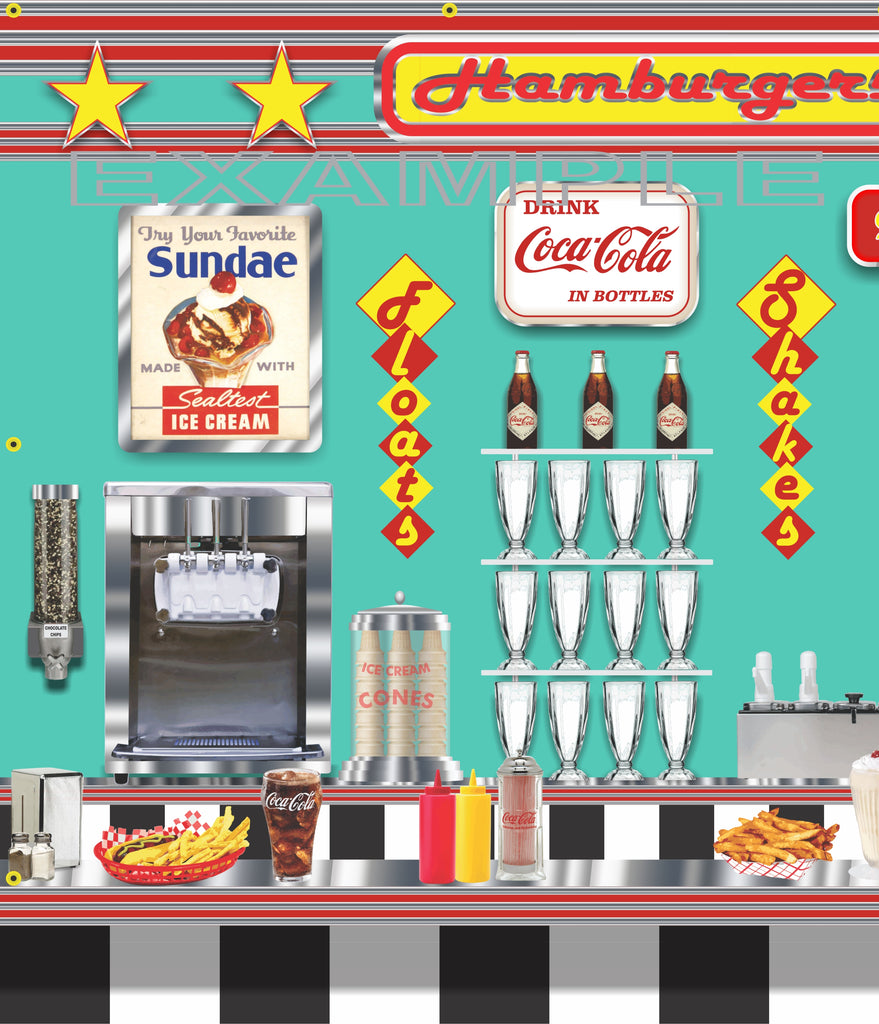This image is a vibrant, digitally rendered depiction of a 1950s-style diner or soda shop. The background features a teal green hue, accented by a red horizontal line outlined in silver near the top, with another red and silver line below. Prominent in the scene are two yellow stars outlined in red. To their right, a sign with a yellow background and a red and silver outline reads "hamburgers" in red cursive font. Below this signage, a milkshake machine and a clear ice cream cone container, labeled "ice cream cones" in red, are displayed.

The counter is populated with various details, emphasizing the diner theme. There are three rows of milkshake glasses, three Coca-Cola bottles above, fries, a cup of Coca-Cola, and bottles of ketchup and mustard. Additional nostalgic signs enhance the ambiance, such as "Drink Coca-Cola in Bottles" and "Try Your Favorite Sundae," indicating the use of Sealtest ice cream. The bright, bold color scheme of yellow and red, alongside the detailed illustrations of classic diner items, collectively evoke the lively atmosphere of a vintage diner.